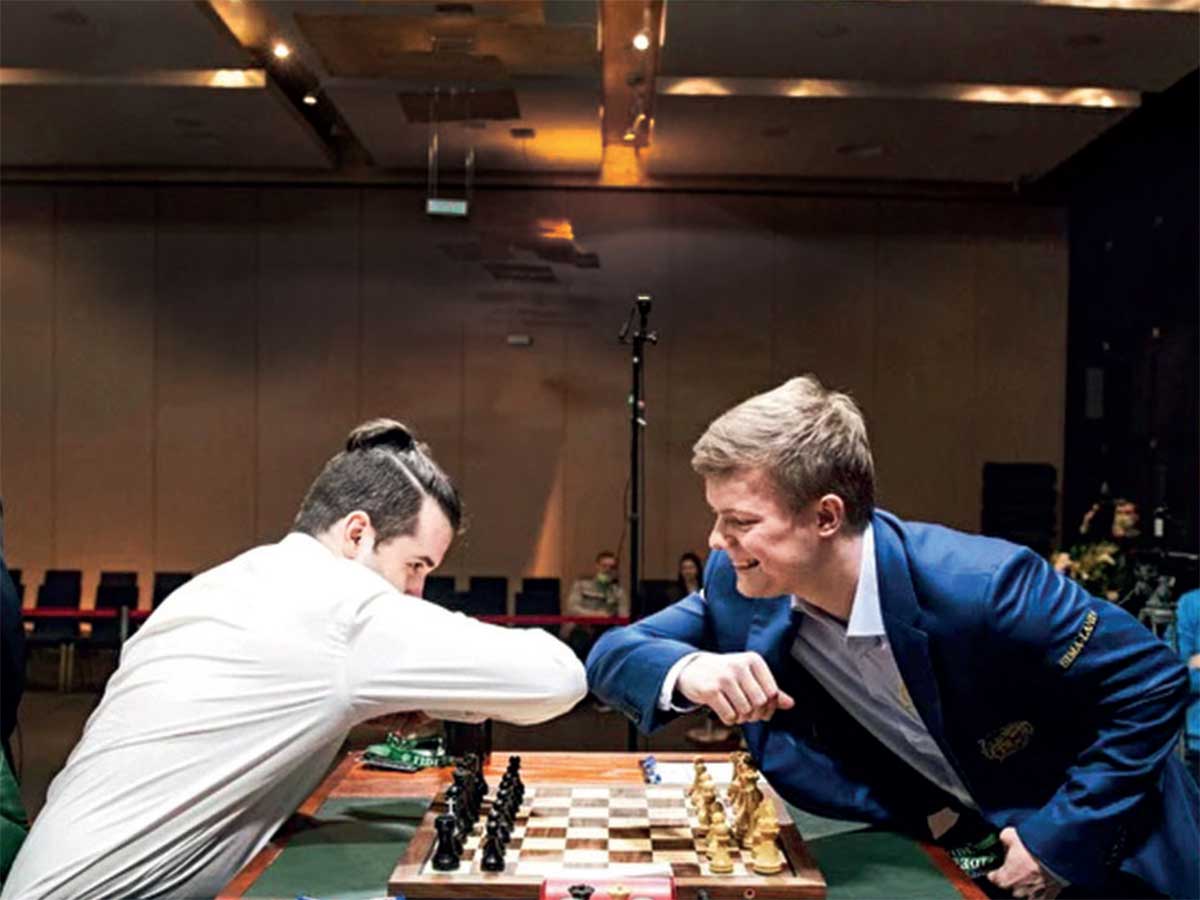In this detailed full-color indoor photograph taken with artificial light, we witness the beginning of a chess match between two young men, possibly during a tournament in an auditorium. Instead of shaking hands, they are bumping elbows, perhaps as a COVID-19 precaution. The man on the left is playing with black pieces and sports a man bun and a long-sleeved white shirt that covers his mouth. The man on the right, playing with white pieces, is a blonde wearing a blue suit jacket over a light blue button-up shirt, smiling openly. They sit at a brown table with a green placemat supporting a chessboard that features brown and white tiles. Behind them, a sparse crowd of three people, including a man and a woman, can be seen amidst rows of chairs, observing the commencement of the game. Overhead lights illuminate the scene, emphasizing the serious yet friendly atmosphere of the competition.